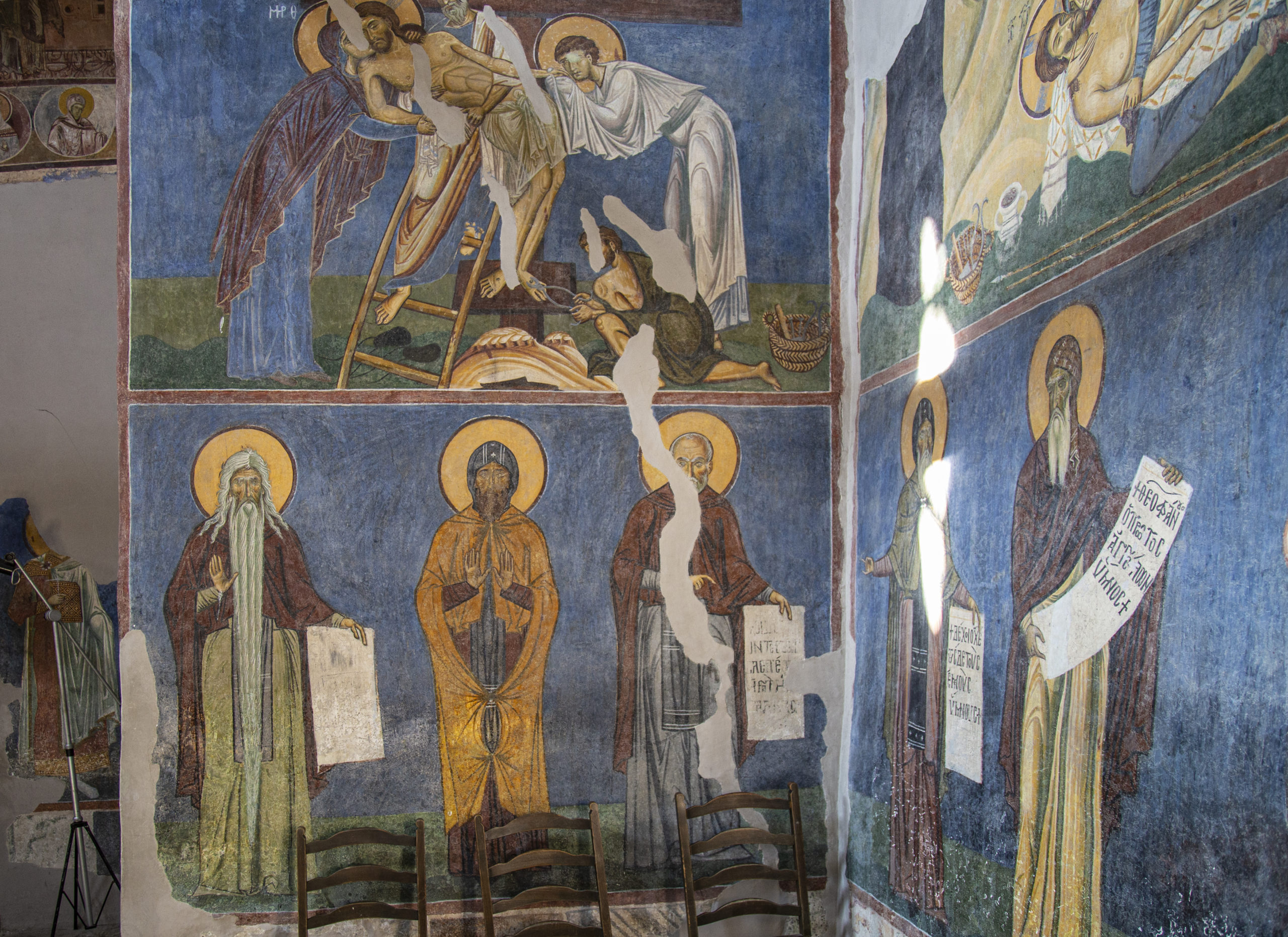This photograph captures an aged, large-scale religious painting or fresco, likely situated inside an old or abandoned church. The artwork, divided into four panels, exhibits noticeable damage with white streaks and tears marring its surface. Each panel features multiple figures, predominantly saints, easily recognizable by the golden halos encircling their heads and shoulders. The backgrounds of these panels consist uniformly of a blue sky in the upper sections and green earth or ground in the lower thirds.

In the upper left panel, a poignant scene unfolds where Jesus is being taken down from the cross. A figure is seen kneeling to remove a nail from His feet, while another, robed in white, holds His hand. The possible Virgin Mary, dressed in blue, cradles Jesus as He is lowered from the cross. Adjacent to this, in the upper right panel, another male saintly figure lies down, seemingly being held by the Virgin Mary, consistent with her blue attire.

The lower panels depict five probable saints dressed in varied colored robes. Four of these figures hold tablets or documents; three tablets bear lettering, while one is notably faded. The fifth saint stands empty-handed. The paintings' muted colors are indicative of their age, and faint glimpses of chairs and objects in the photograph's foreground suggest the presence of seating or furnishings typically found in a church setting.